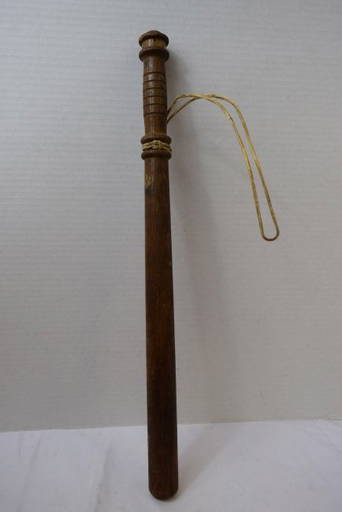The photograph, vertically oriented in a rectangle shape, features a dark wooden club leaning against a faintly striped, light beige wall. It sits on a white surface, casting a shadow on its right side. The club, resembling a long, tapered stick rather than a baseball bat, has a handle adorned with several wooden rings and horizontal ridges. A piece of natural-colored, yellowish twine is looped around the handle, extending to the right side of the image. The thick, rounded bottom of the club rests firmly on the white surface, creating a stark contrast with its darker shade and textured background.